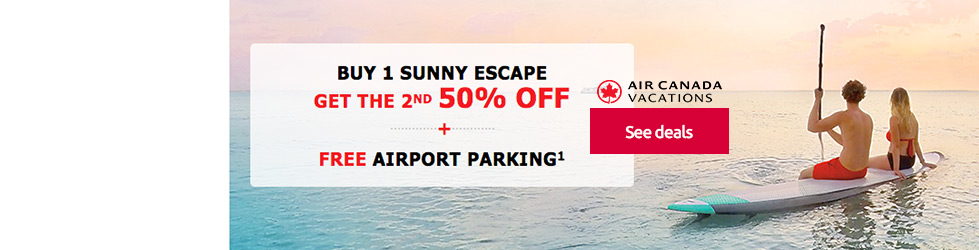This advertisement banner from Air Canada Vacations features a picturesque scene aimed at enticing travelers to book a sunny getaway. The promotional text prominently displays an offer: "Buy one sunny escape and get the second 50% off, plus free airport parking." A prominent red button beneath the text invites viewers to "See Deals."

Complementing the offer, the background image showcases a serene moment of a couple paddleboarding on the ocean at either sunrise or sunset. The sky is painted in varying hues of pink, blending seamlessly into the cyan blue water. The couple, facing away from the camera towards the horizon, creates a sense of togetherness and adventure. The man, positioned at the center of the gray paddleboard with a blue tip, is donning red swim trunks, while the woman sits to his right in a black and red swimsuit. He has black hair, whereas she sports blonde hair with dark roots. The calm and inviting scene vividly conveys the allure of a romantic vacation getaway.